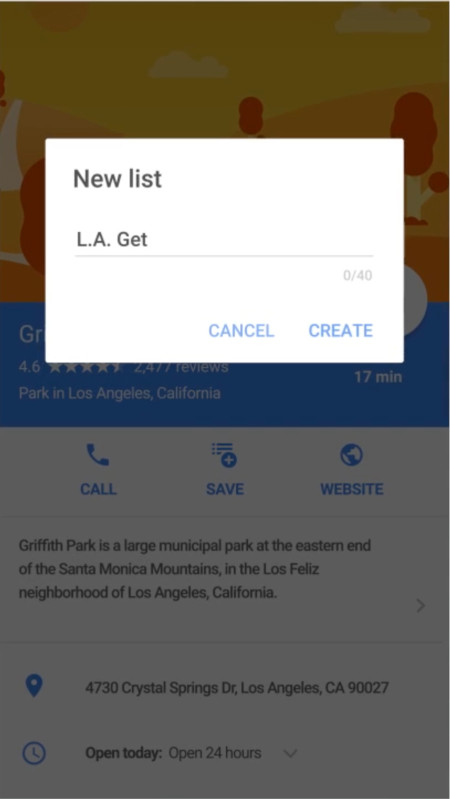In the foreground of the image, there is a set of menu options labeled: "New List," "LA," "Get," "Cancel," and "Create." Positioned prominently in the background is a 4.6-star rating based on 2,477 reviews. The text indicates that the location is Griffith Park, a large municipal park at the eastern end of the Santa Monica Mountains, nestled in the Los Feliz neighborhood of Los Angeles, California. Specific location details such as the address—4730 Crystal Springs Drive, Los Angeles, California, 90027—are provided. The park is described as being open 24 hours a day. The image features a color palette of orange, yellow, black, and blue set against a white background.